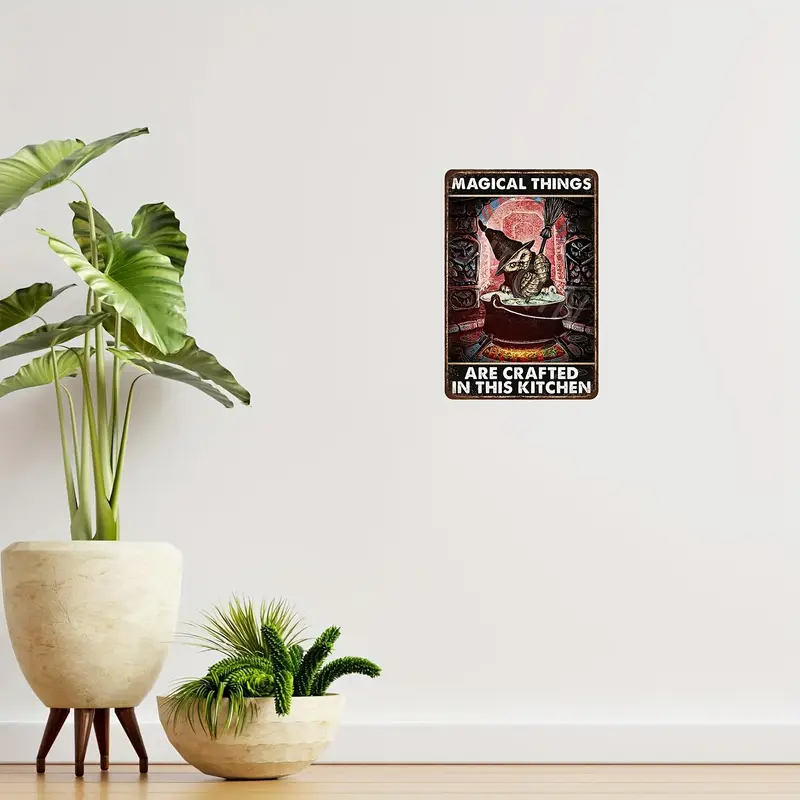The full-color, square photograph depicts a carefully staged indoor scene, illuminated with natural light. The setting features a plain gray wall above a light beige wood floor. At the point where the wall meets the floor, a running board is visible. Positioned on the floor are two potted plants: the one on the left is a tall palm plant with large leaves, housed in a planter raised on a wooden stand, and the one on the right is a low bowl containing a spiky green cactus. Affixed to the wall is an artistic sign with black background and white text, featuring an owl in a pointed witch's hat, stirring a cauldron with a broom. The sign reads "Magical things are crafted in this kitchen."